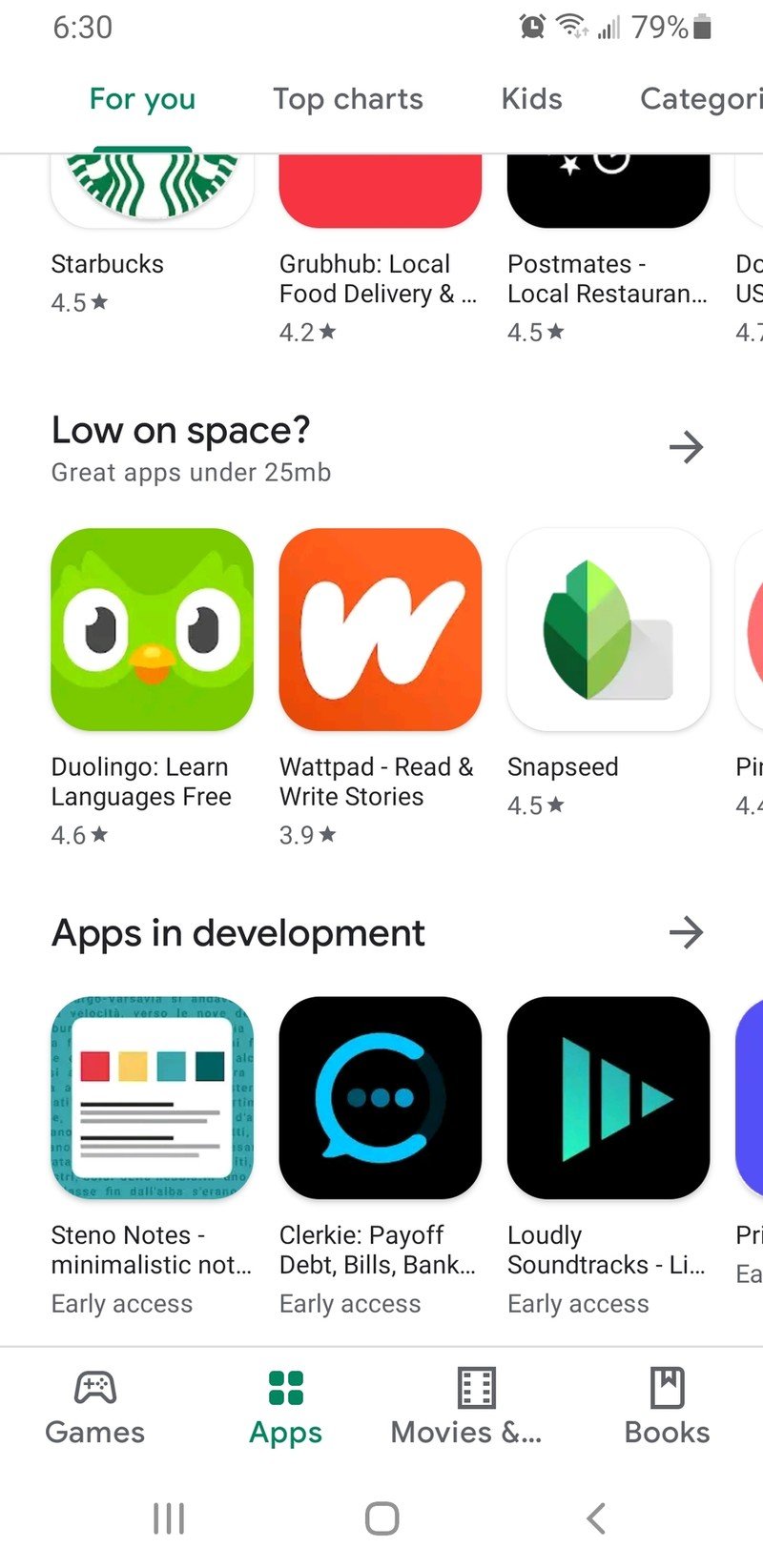A detailed image caption can be written as follows:

---

The screen capture features a mobile phone's app store interface with a white background. The top status bar indicates the time as 6:30 AM (or PM) on the upper left-hand corner and the battery level at 79% on the upper right. The header section of the app store displays tabs labeled 'For You,' 'Top Charts,' 'Kids,' and 'Categories,' although the latter is partially cropped, displaying only 'Categorie.' The 'For You' tab is selected, displaying curated app recommendations.

Below the header, the first row showcases individual app listings: 'Starbucks' rated 4.5 stars, 'Grubhub' rated 4.2 stars, and 'Postmates' Local Restaurants rated 4.5 stars, although the fourth app in this row is partially cut off by the screen's edge.

Scattered through the page is a section titled 'Low on Space? Great Apps under 25 MB,' featuring a variety of apps. The visible apps include 'Duolingo' rated 4.6 stars, 'Wattpad' Read and Write Stories at 3.9 stars, and 'Snapseed,' which boasts a 4.5-star rating. The fourth app in this section is also clipped by the screen. At the bottom of the screen, partial icons of apps indicate there are more suggestions that are cut off.

---